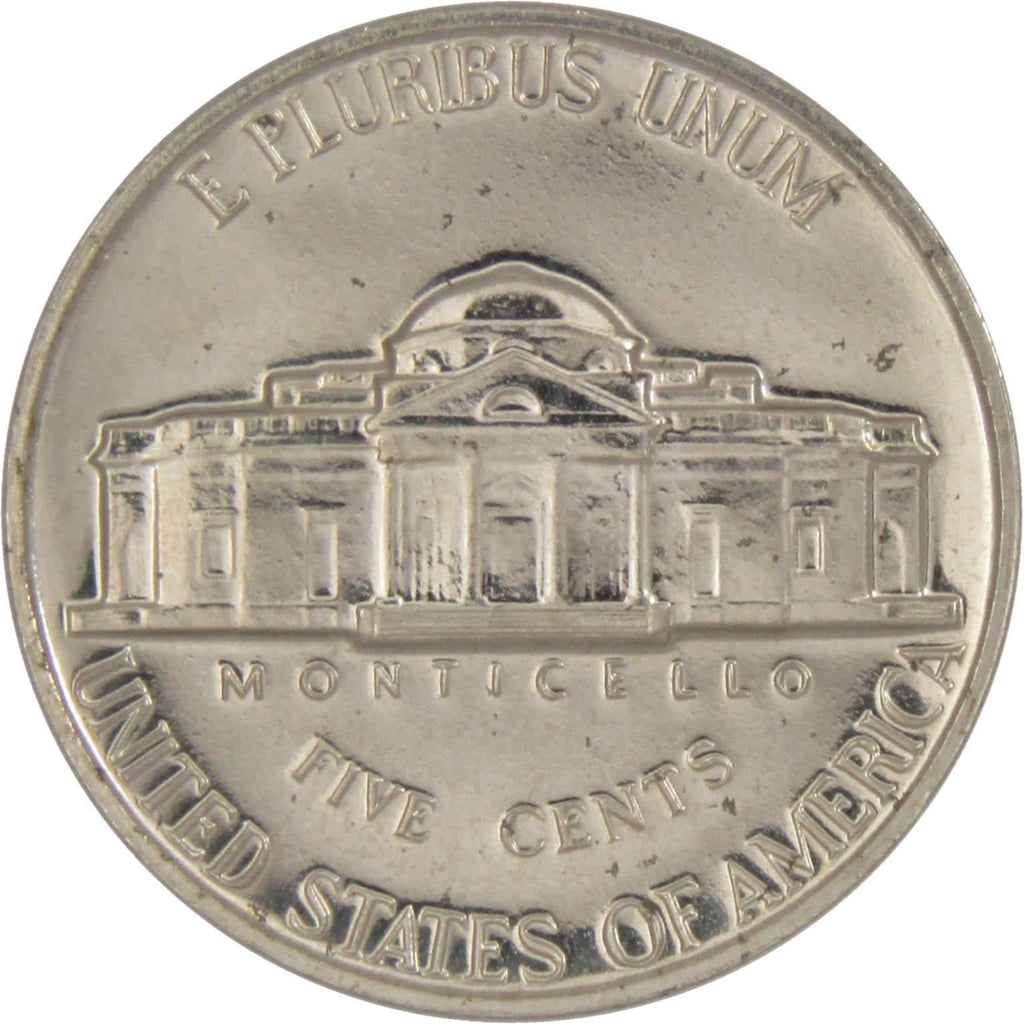This image is an extreme close-up of a somewhat worn, silver-colored U.S. nickel, taking up the entire frame against a solid white background. The coin’s rim forms a slightly darker, thin border around its edge. At the top, curving along the inner edge, the text "E PLURIBUS UNUM" is displayed in all capital letters. In the center, there is an image of Monticello, which is labeled "MONTICELLO" just below the building in all caps. Further down, "5 CENTS" is spelled out, with "UNITED STATES OF AMERICA" curving along the bottom edge, also in all caps. The overall shading of the coin varies due to its reflectiveness, highlighting its worn but not excessively old condition.